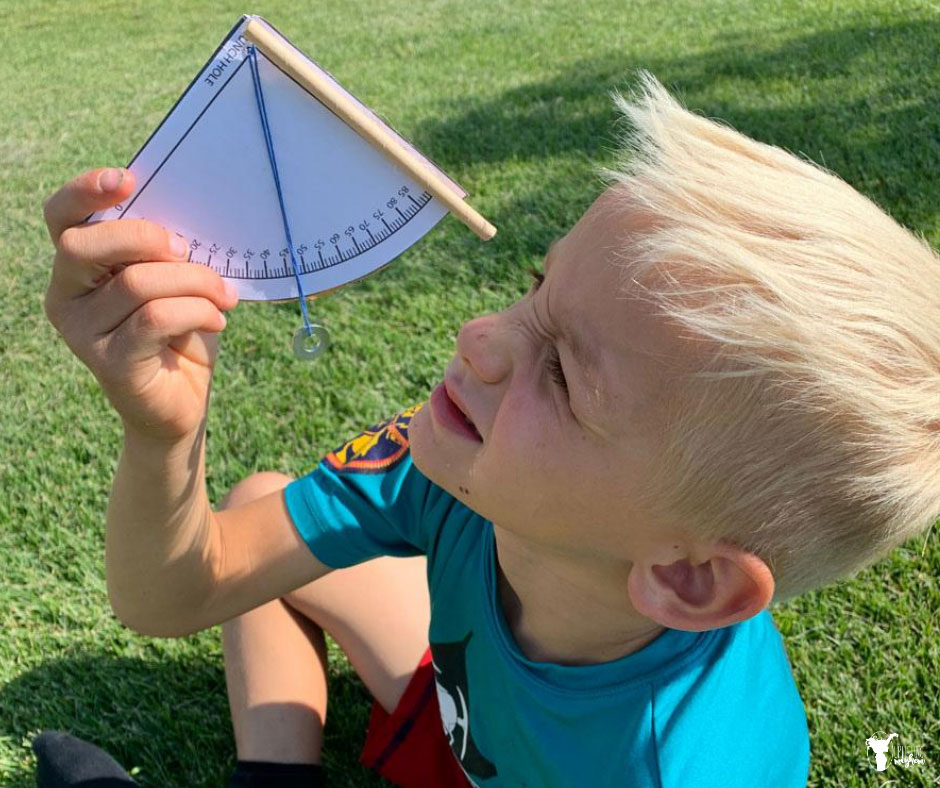In this detailed image, a young Caucasian boy, likely aged six to eight, is sitting cross-legged on sunlit grass, absorbed in a scientific experiment involving a homemade quadrant. The boy has short blonde hair and is wearing a turquoise blue shirt, adorned with a patch on his right sleeve, and red shorts complemented by black socks. He is intensely focusing on a white quadrant made from a thin cardboard tube and a quarter-circle cut-out of paper. Attached to the quadrant are two small sticks, and it features black degree markings on the white paper. A string, with a metal bob at the end, hangs down from the center of the quadrant, angled slightly less than 47 degrees. The boy squints as he holds up the quadrant, likely to measure the angle of the sun. The backdrop includes more grass and the shadow of a tree, suggesting the scene is set in a sunny yard.